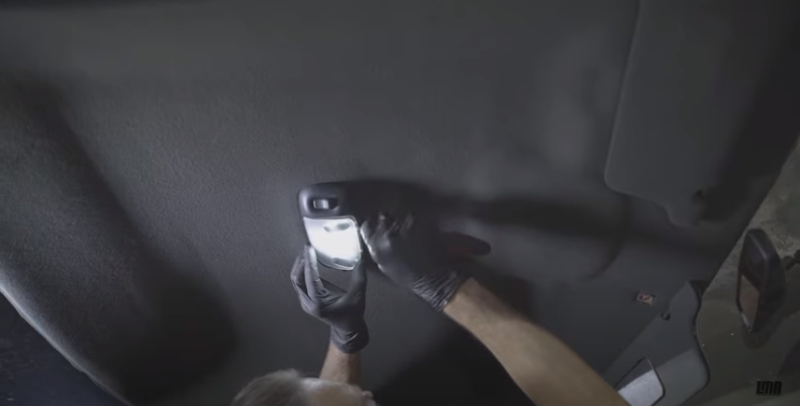The image features a dark, textured fabric backdrop, covering a wall with two prominent protrusions on the left and right sides. Positioned centrally, a person's head and arms extend from the background, with their hands clad in black latex gloves. In their left hand, they grasp a sleek, black device with a screen and a rotating button at the top. A distinctive shadow of the device is cast on the wall behind. A thick, curved line runs from a sizable object on the right, bending towards the man's hands. The individual’s hair is slightly visible. To his side, an additional black device is mounted on the wall, accompanied by a dark gray plastic component beneath it. The bottom right corner of the image features the text "UNA."